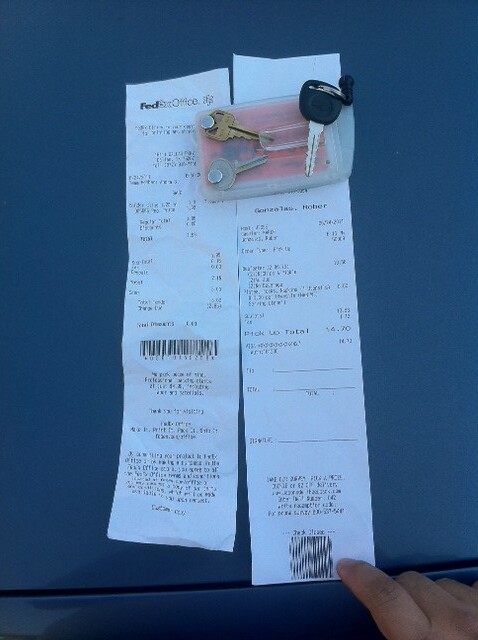This image depicts two lengthy receipts from a Federal Express office. The first receipt prominently features a barcode and detailed transaction information, indicating a purchase has been made. Adjacent to it lies a second, even longer receipt, which is being pressed down by a human hand. The scene appears to be set on the hood of a blue-gray car. Atop the second receipt, car keys rest, comprising a gold key and a silver key, which are placed within a transparent square container. Notably, a red object is visible inside the container, seen through its clear sides.